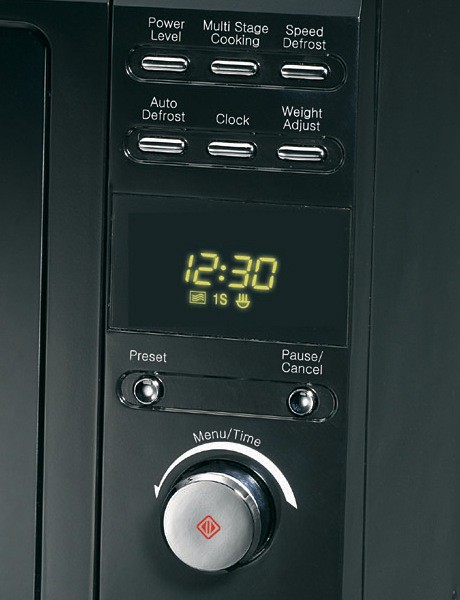The image shows a detailed close-up of a black microwave oven's operating panel. At the center, there is a digital clock displaying the time "12:30" in bright yellow digits. Surrounding the clock are various functional buttons, including "Preset," "Pause," and "Cancel." Below these buttons is a manual timing dial for precise control.

At the top of the panel, there are six additional buttons: "Power Level," "Multi-Stage Cooking," "Speed Defrost," "Weight Adjust," "Clock," and "Auto Defrost," each clearly labeled for ease of use. Notably, the "Timer" button features a distinctive red diamond logo with a smaller red image in its center, which might hint at the brand or manufacturer of the microwave, although no explicit branding is present elsewhere in the image.